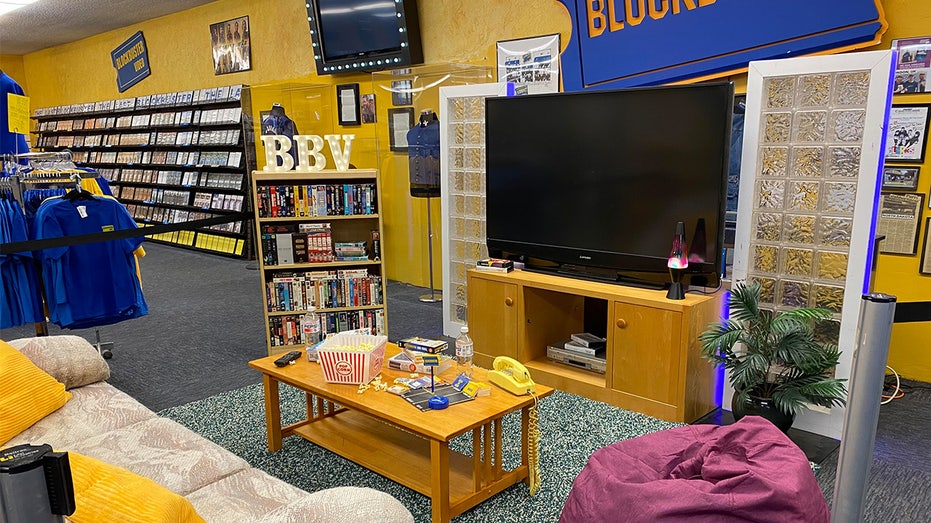This detailed, color photograph depicts a nostalgic living room setup inside a Blockbuster video rental store. Dominated by a retro ambiance, the scene features a large television centrally positioned, surrounded by shelves filled with DVDs and a rack of blue t-shirts. The living room area includes a cozy couch located on the bottom left, in front of a wooden coffee table adorned with an old school landline phone, a remote, board games, and a bowl of popcorn. A beanbag chair and a pot plant add to the homely atmosphere. The walls are vibrantly painted in yellow, embellished with blue signs bearing the iconic Blockbuster logo. Additional elements include picture frames, a lava lamp, and a shelf containing more movies, enhancing the nostalgic charm of this indoor setup.